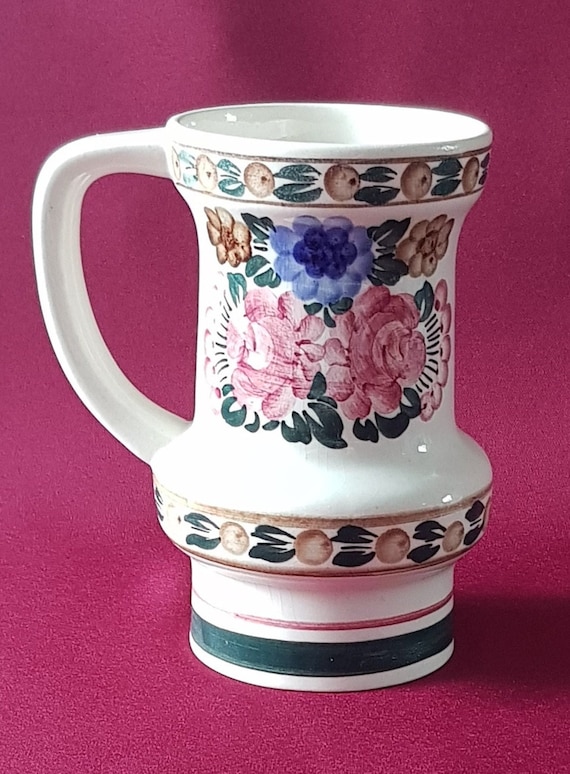This image captures a vintage ceramic mug, notable for its unusual shape: it flares outward at the bottom before curving back into a narrower base. The mug features an ornate design with floral motifs, including beige, pink, and blue flowers accompanied by green leaves. The handle is large and prominent, adding to its distinctive appearance. The mug's background is a rich fuchsia or hot pink color, matching both the surface it rests on and the backdrop. At the top and bottom of the wider section, there are repeating plant-like patterns, and the base showcases alternating green and thin reddish-pink stripes against a white background. The overall look is reminiscent of both a coffee mug and a beer stein, but with decorative elements that suggest it might not be intended for everyday use.